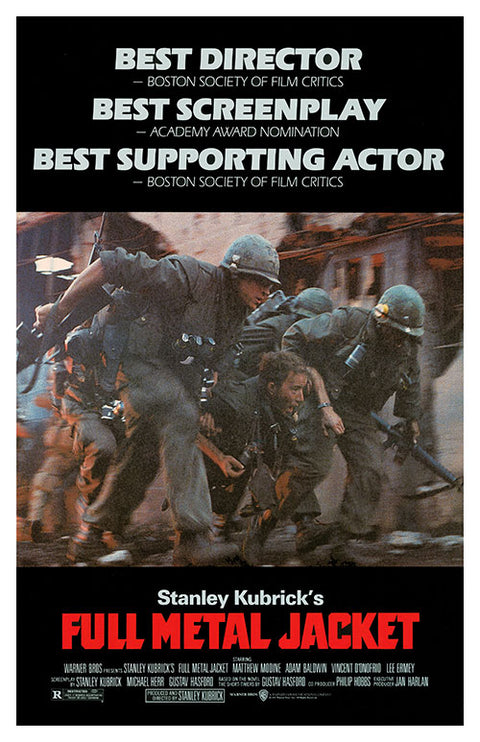**Movie Poster for "Full Metal Jacket"**

At the top of the poster, prestigious accolades are highlighted, including:
- Best Director by the Boston Society of Film Critics
- Best Screenplay, which received an Academy Award nomination
- Best Supporting Actor by the Boston Society of Film Critics

Below these accolades, a dynamic screenshot from a pivotal scene in the movie is featured. This scene captures men in military attire forcefully pulling another man between them. Notably, the pulled man lacks a helmet, while the others wear theirs, adding a layer of tension and immediacy to the image.

Centered below the action shot, bold red text announces "Stanley Kubrick's Full Metal Jacket." Additional details about Warner Brothers, the film's cast, and other production credits are listed beneath the title.

The poster's overall color scheme is a stark black, with white font used at the top for text, and "Full Metal Jacket" standing out in red. The central image maintains a gritty, muted color palette, enhancing the raw, live-action feel of a major scene from the movie.